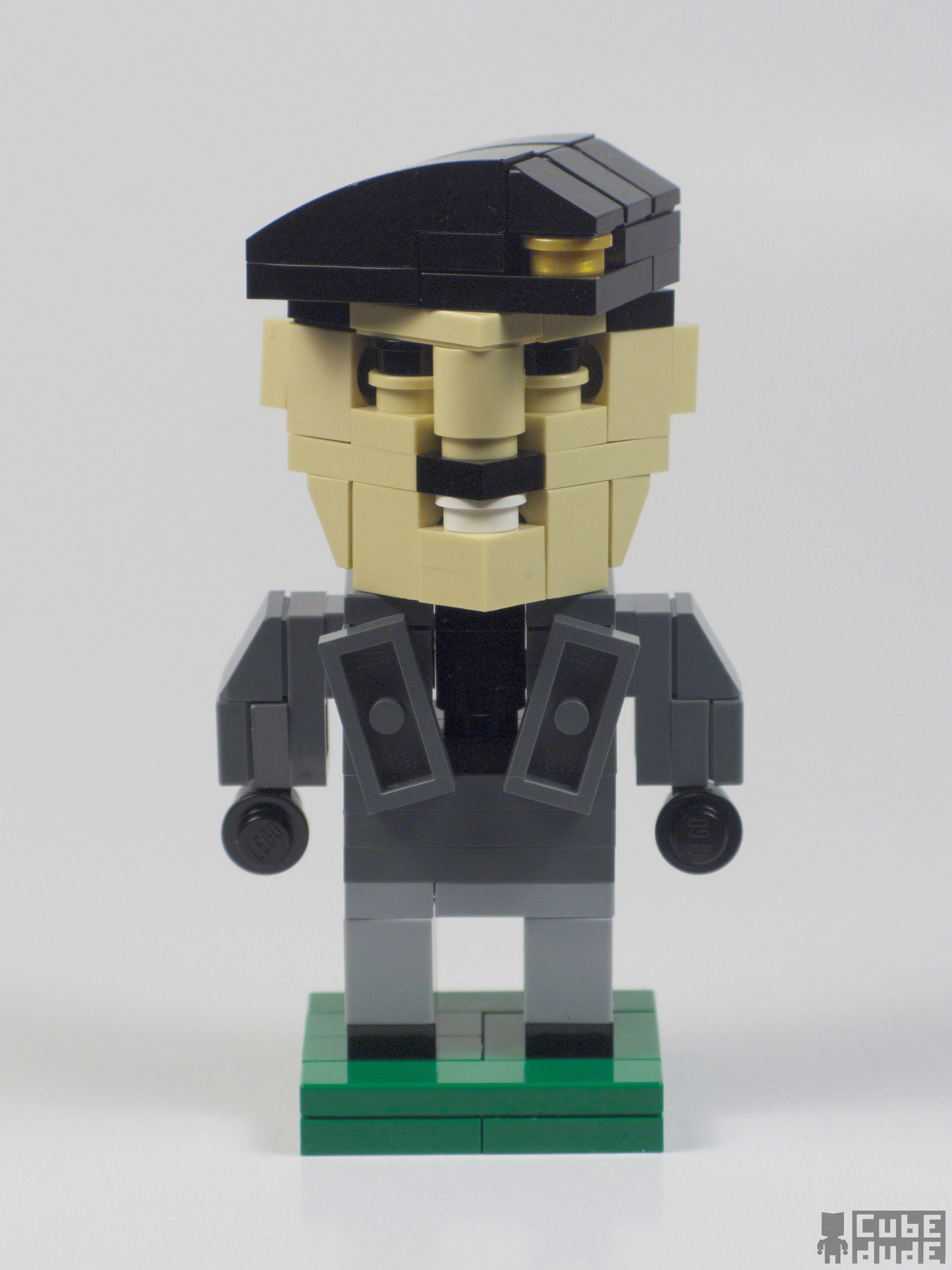The image depicts a detailed Lego figure referred to as a "Cube Dude" situated centrally on a green platform, representing the ground. The figure appears to be a man with fair skin, characterized by a distinct black mustache, thick eyebrows, and a visible set of teeth. He is dressed in a gray long-sleeve shirt and gray pants, complemented by black shoes and black gloves or hands. Enhancing his attire, he wears a black beret featuring a gold accent. The backdrop of the image is predominantly gray and white. In the lower right corner, there is a gray logo depicting a block figure with the text "Cube Dude" clearly displayed against the gray background. The setting suggests that the Cube Dude is positioned on a table.